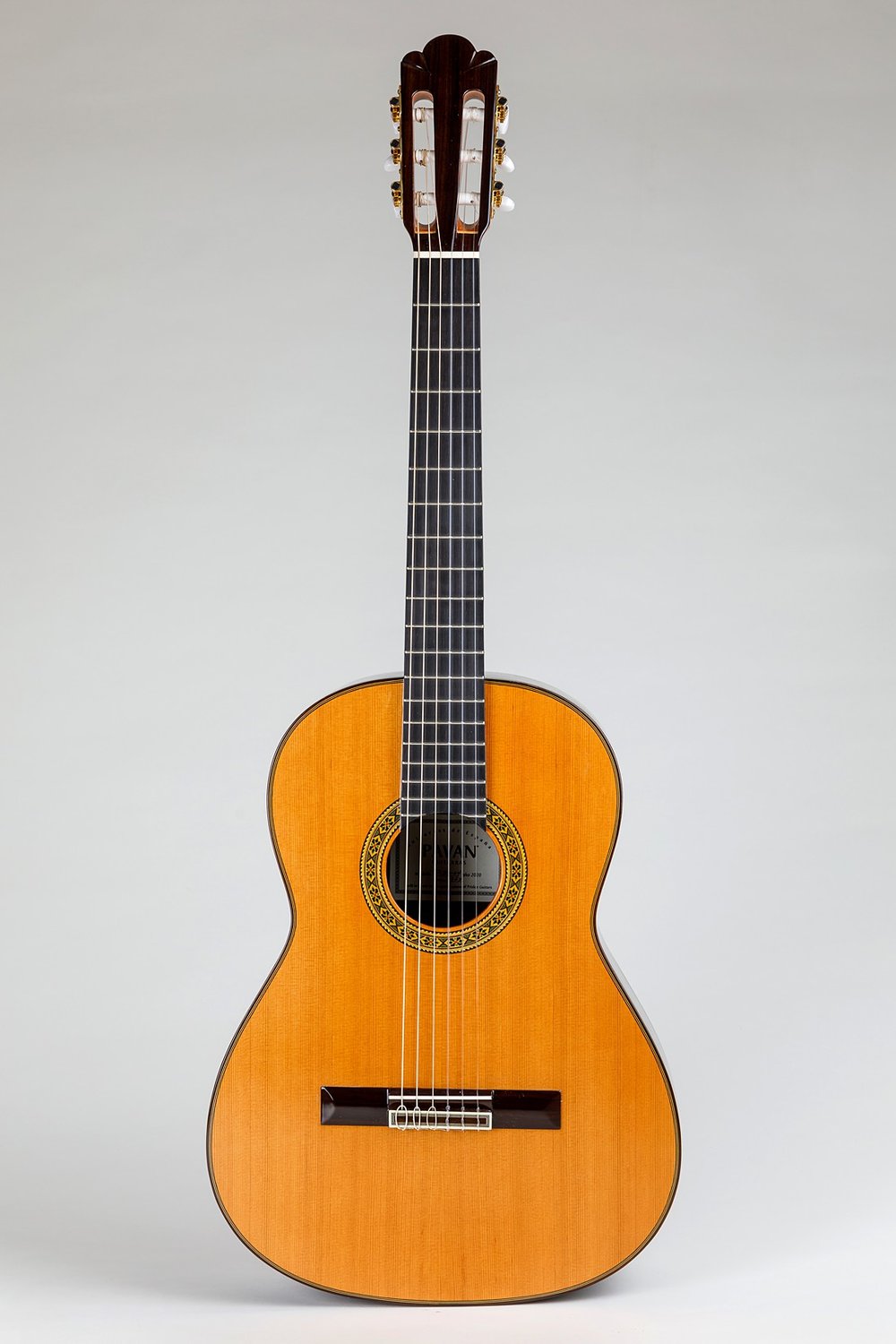This image showcases an acoustic guitar standing upright against a gray-black background. The guitar's body features a medium brown wood finish, prominently displaying its natural wood grain. The instrument is viewed from the front, with its base resting on the ground and its neck pointing upward. Six white nylon strings stretch vertically from the top of the guitar to the bridge. Notably, around the central sound hole, there's an intricate yellow-brown inlay with a pattern reminiscent of Aztec designs, adding a touch of artistry to this otherwise traditional-looking acoustic guitar. The background is solid and unobtrusive, ensuring the focus remains solely on the guitar.